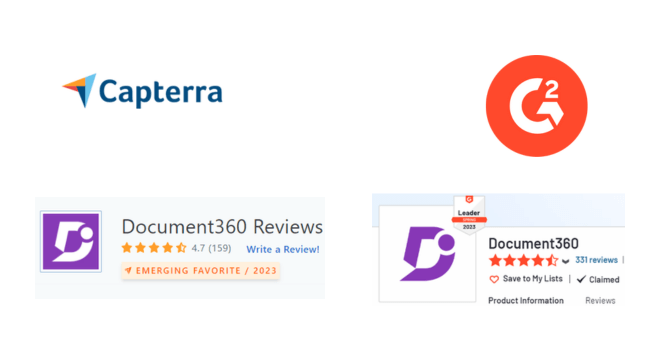This image is a screenshot of a minimalist advertisement or pop-up ad for a software review website. The background is entirely white. In the top left corner, the brand name "Capterra" is prominently displayed in royal blue, accompanied by its logo, which features an arrow pointing upwards and to the right. The arrow is colorfully segmented with light blue, yellow, red, and dark blue sections.

In the top right corner, a circular orange logo with a white "G2" signifies a different related service or product.

Beneath the "Capterra" heading, there's a text section labeled "Document 360 Reviews." This section includes a purple rectangle enclosing a white "D" and indicates a high rating of 4.7 stars. Directly below this, the label "Emerging Favorite (2023)" is displayed in orange. A light blue "Write a Review" link appears right below.

To the right of this, next to the "G2" logo, is another purple "D" logo on a white background, which reverses the color scheme of the earlier logo. Next to it, the name "Document 360" is mentioned again, this time alongside a note of "331 reviews" written in blue and an approximate 4.5-star rating with stars in orange.

Underneath, there are options "Save to My Lists" featuring a heart icon, followed by a check mark and the word "Claimed," indicating that the product or service has been authenticated. At the bottom of this section, "Product Information and Reviews" is displayed in a gray font.